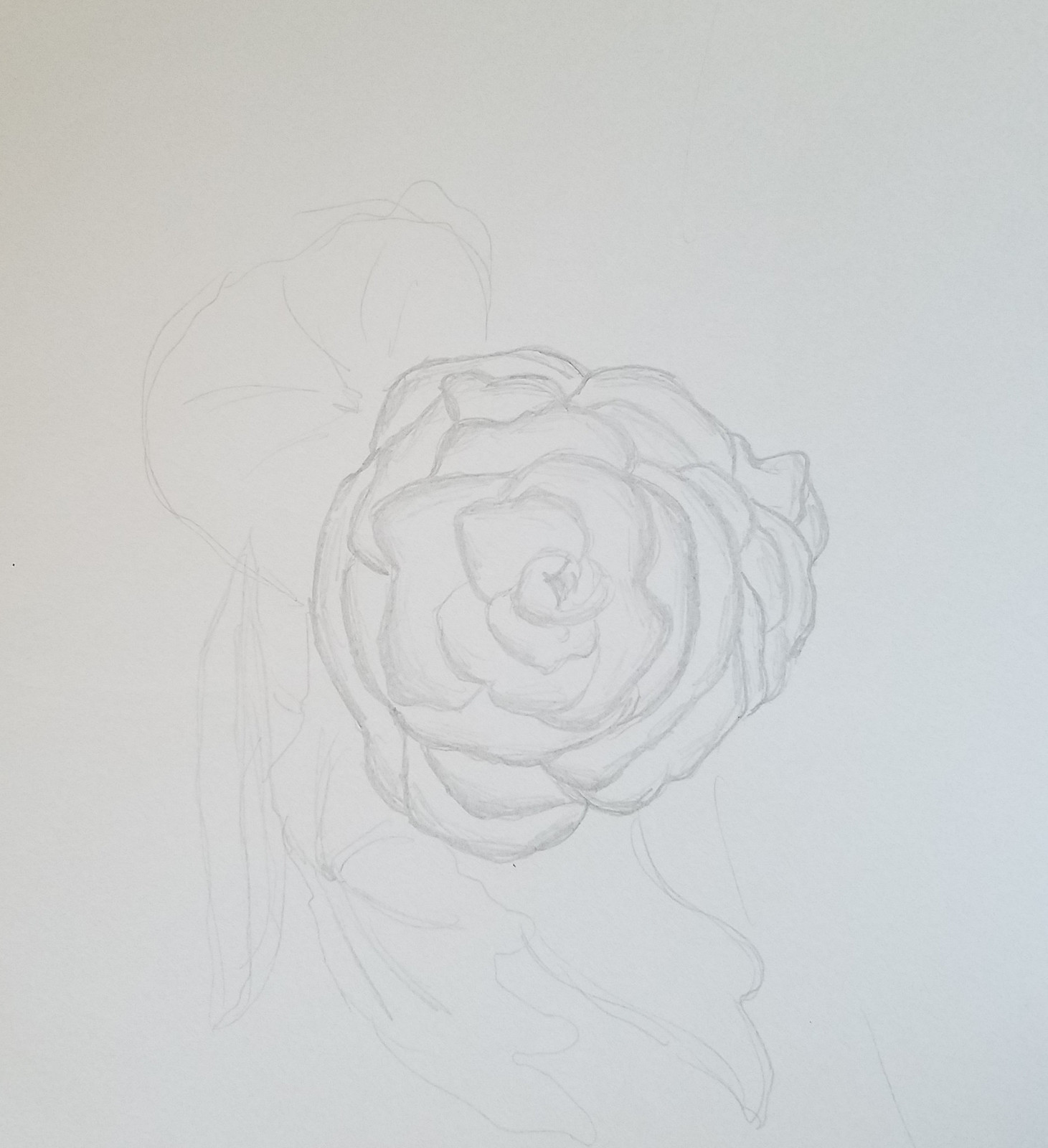This is a highly detailed pencil sketch on a white piece of paper, focusing on an intricately drawn flower head that appears to be a rose. Viewed from above, the rose features multiple layers of petals, each thoughtfully shaded to provide depth and character. The center of the rose is prominent, surrounded by thick, well-defined petals. Lightly sketched lines and markings around the flower suggest parts of a stem and leaves or possibly preliminary guidelines that the artist hasn’t fully developed. There is no text or artist's signature in the image. In the background, faint and unclear pencil marks resemble a poorly drawn figure with an oddly shaped head and arms, possibly an erased figure or something showing through from the back of the paper, but the dominant and most detailed aspect is unmistakably the rose at the center.